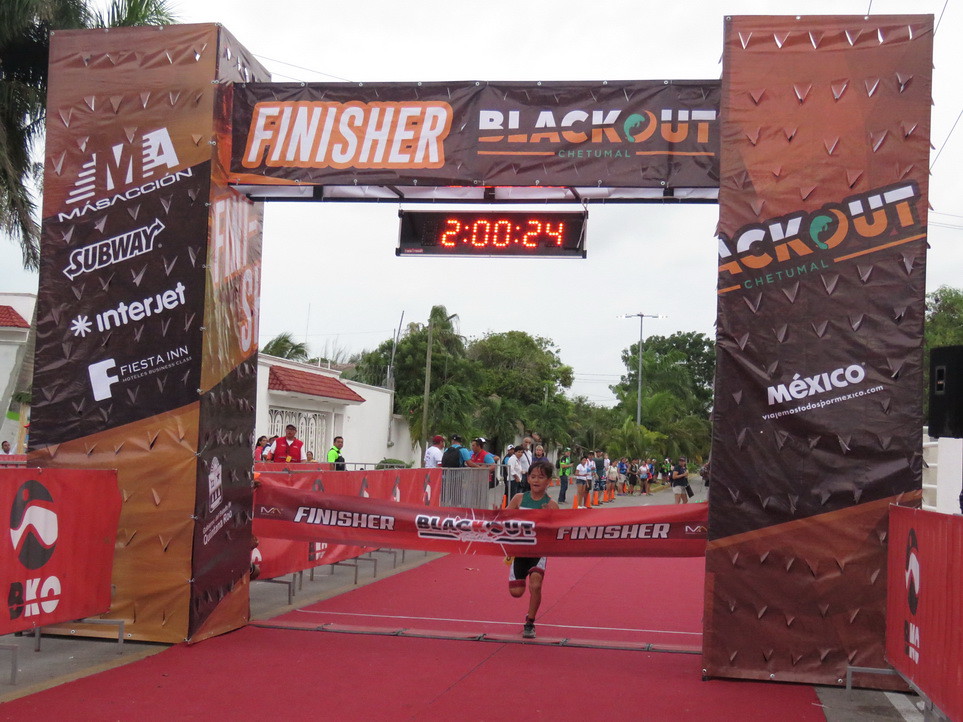In this outdoor image of a marathon finish line, a young boy is on the verge of crossing and tearing through a banner. The banner prominently displays "Finisher, Blackout, Finisher" in orange and white font, with hints of green, and is part of an arch structure marking the race's end. Above the finish line, there is a digital clock showing "2:00:24", indicating the elapsed time. The archway also features text reading "Finisher, Blackout, Chetumal" at the top, along with "Mexico" on the right side. On the left side, several sponsor logos are visible, including Massassion, Subway, Interjet, and Fiesta Inn. Spectators are lined up behind gates and cones on both sides of the street to witness the event. The arch and surrounding banners all contribute to the vibrant atmosphere of the marathon, likely taking place in Mexico, with evidence from the website "ViajamosTodosPorMexico.com" displayed.